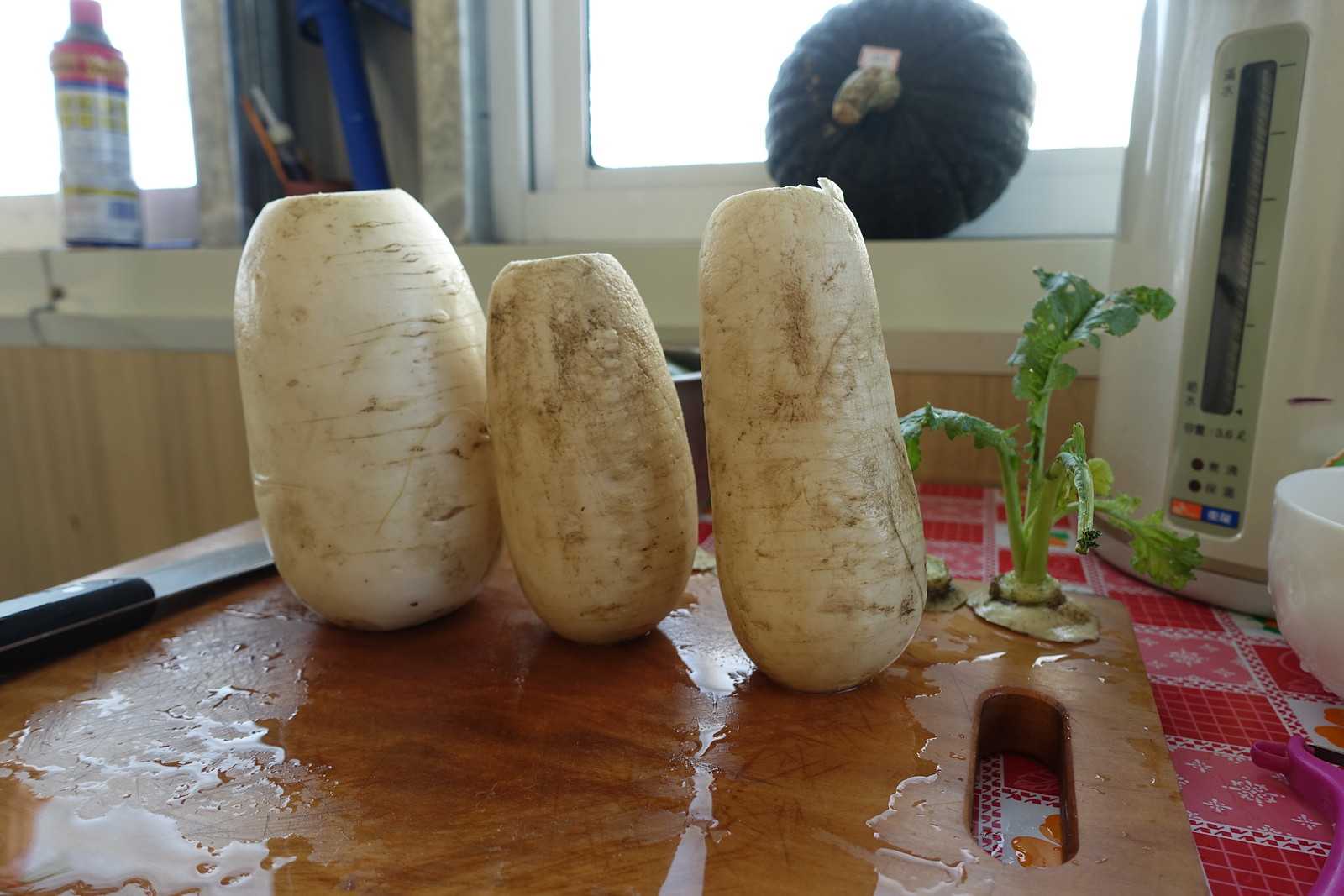This vibrant photo, taken inside a cozy kitchen, centers on a wooden cutting board sprinkled with water droplets. Three white, root vegetables, possibly turnips or daikons, stand upright with their tops and bottoms sliced off. To the left of the vegetables, a knife with a wooden handle lies flat, while to the right, one of the leafy vegetable tops sits prominently. The cutting board rests on a red and white checkered tablecloth adorned with small white flowers. 

In the background, two windows framed by a wooden wall draw attention. The right window, which sits directly behind the vegetables, features a round green squash perched on the sill. The left window is partially visible, revealing a blue bottle with a colorful, predominantly white, yellow, and red label. Additionally, a white kitchen appliance with red and blue buttons and a white bowl sit on the table. The overall image reflects a casual, homey atmosphere with a hint of culinary activity.